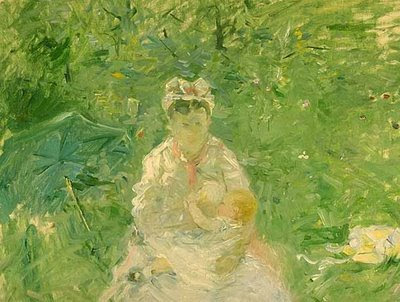In this oil canvas painting, the central focus is a woman with brown hair, wearing an old-fashioned bonnet and a pink, white, and gray outfit, possibly a dress or long robe. She is kneeling or sitting in a lush, green grassy area, surrounded by a hazy, green-hued outdoor backdrop that vaguely suggests trees. The woman is tenderly holding a baby, who is feeding at her breast. The baby has short blonde hair, is dressed in a little dress with black shoes, and also appears to have a red scarf around its neck. To the left, there is the faint, green shape of an umbrella. The overall composition is enveloped in shades of green, lending a tranquil and pastoral atmosphere to the scene.